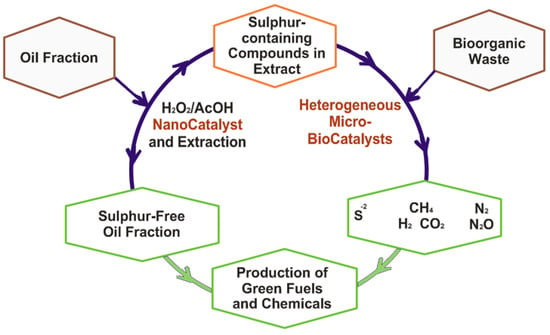This image is a detailed diagram illustrating a chemical process. The focal point is a central circle, half-blue at the top and half-green at the bottom, labeled "Sulfur Containing Compounds in S Extract." Radiating from this central circle are various geometric shapes connected via colored lines indicating the flow of the process.

On the top half of the circle, a blue section leads to a label "Bio-organic Waste" enclosed in a brown box, from which a blue arrow extends to a green box listing chemical formulae such as S², CH₄, H₂, CO₂, N₂, and N₂O. Following the pathway, this leads to another green box labeled "Production of Green Fuels and Chemicals," which then points to "Sulfur-Free Oil Fractions."

The process continues with a green section indicating a separation into an area labeled "Oil Fraction." Within the central circle, details include "H₂O," "ACOH," "Nanocatalyst," and "Extraction" on one side, while on the other side, it labels "Heterogeneous Microbiocatalyst."

The diagram comprehensively maps out the transformation from sulfur-containing components to sulfur-free oil and the production of green fuels, integrating various chemical elements and biological processes.